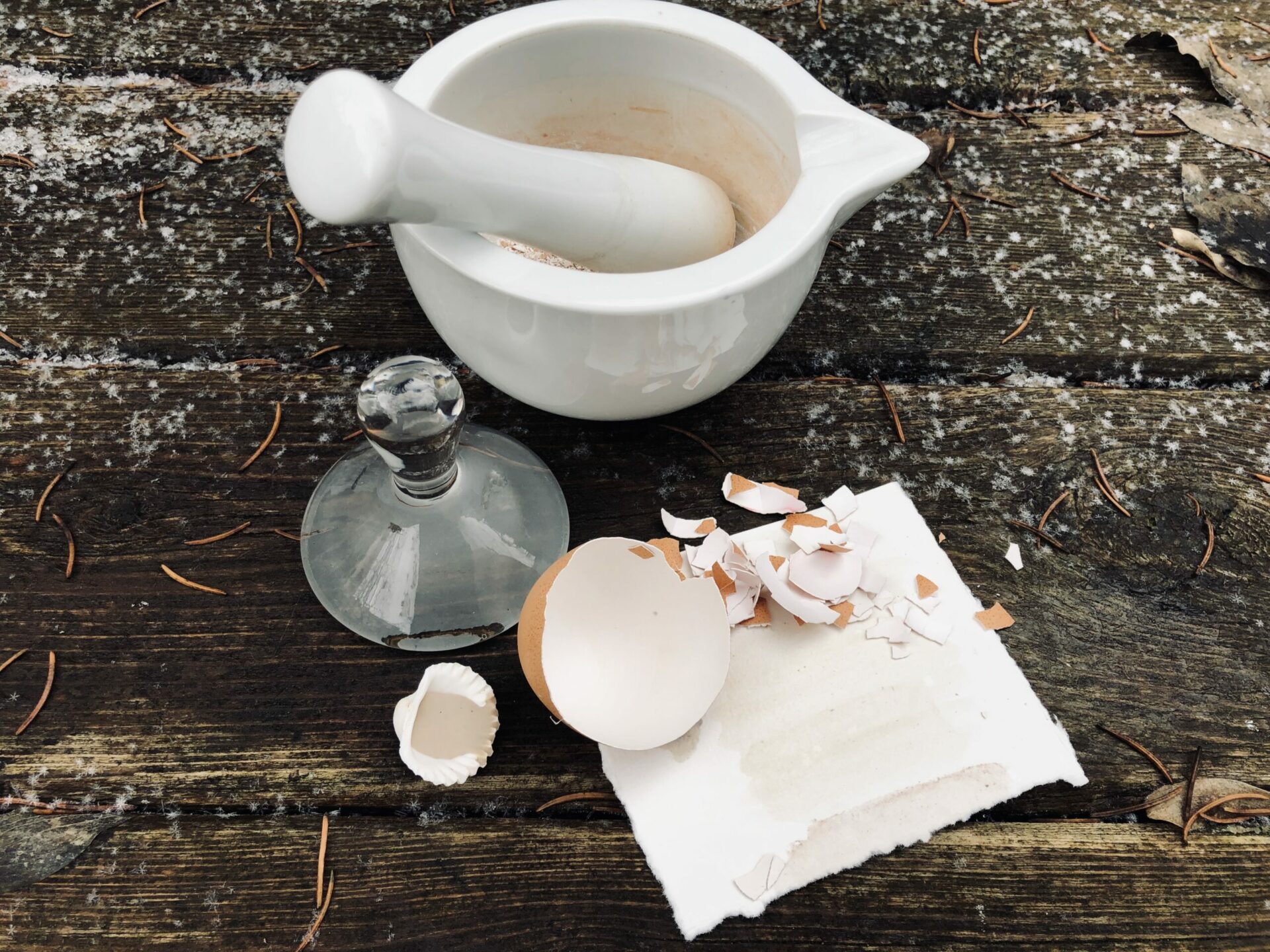On a rustic, dark wooden table lightly dusted with snowflakes, sits a collection of intriguing items. Central to the image is a white ceramic mortar and pestle, which seems to be used for grinding. Beside this set, there is a glass lid, or perhaps a container, with a silver rim. Below these items, a half-broken eggshell rests on a white linen napkin, with small fragments scattered around. The arrangement suggests a kit possibly used for grinding eggshells or herbs, as there are hints of rosemary or another herb inside the mortar. Additionally, there seems to be a white flower adjacent to the eggshell, adding an element of delicacy to the scene.